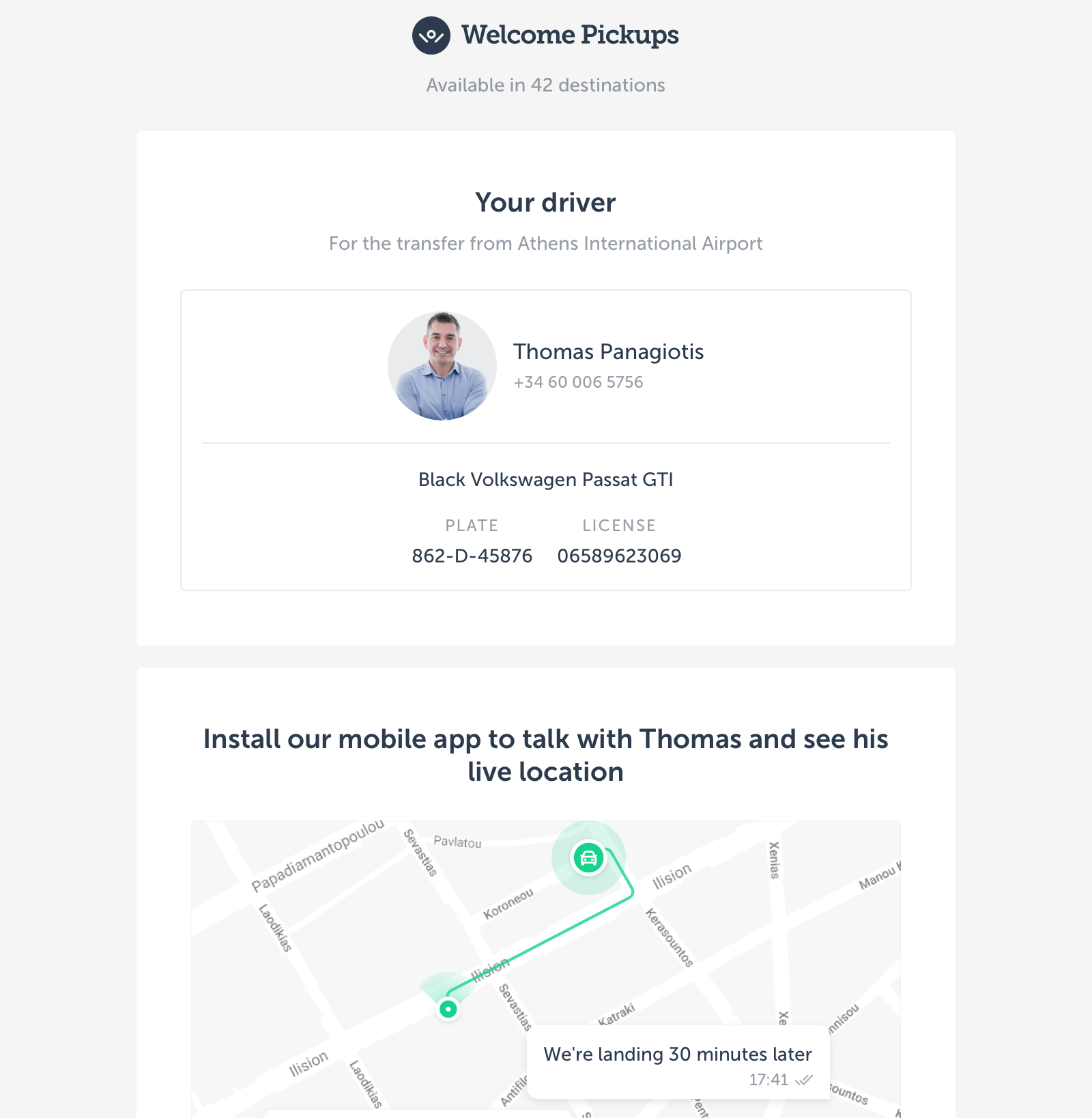This is a detailed screenshot from a webpage or web app. Displayed centrally at the top of the page is a light gray header featuring the "Welcome Pickups" logo alongside text indicating the service is available in 42 destinations. Below this, a prominent white box contains information about your designated driver for a transfer from Athens International Airport.

A circular photo showcases the driver, a man named Thomas Panagiotis, wearing a blue collared shirt. Below his picture are Thomas's contact details and vehicle information. His phone number is listed as +34600065756. Thomas drives a black Volkswagen Passat GTI, with license plate number 862-D-45876 and vehicle identification number 06589623069.

Further down, there is a prompt to install a mobile app, which would allow you to communicate directly with Thomas and track his location. Accompanying this is a small map displaying the car’s route, highlighted by a green line leading to the destination marked with a green dot. Additionally, there is a timestamped message visible in the interface: "We're landing 30 minutes later," sent at 17:41 (or 5:41 PM).

The main focus of this screenshot is providing comprehensive information about the driver, vehicle, and real-time location details to ensure a smooth and coordinated transfer from the airport.